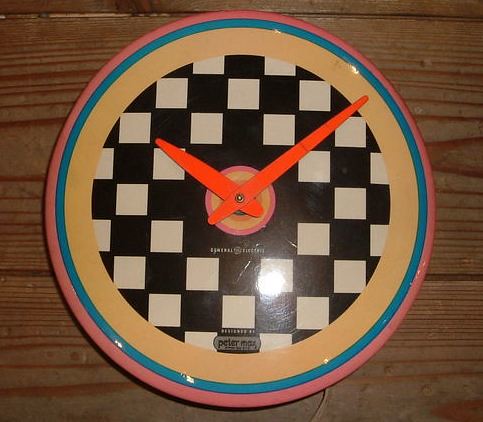In the image, a round clock is centrally positioned against a square, wood-textured platform with a rich brown hue. This platform serves as the backdrop for the clock, enhancing its visual appeal. The clock itself features a series of concentric borders: the outermost is a vibrant pink, followed by a striking blue, and then a warm tan border. The innermost section of the clock showcases a black and white squared pattern, creating a dynamic background. At the very center of the clock's face, there is an inscription in white text, although it is too small to be legible. The intricate details and varied colors contribute to the clock's aesthetic, making it a visually engaging subject.